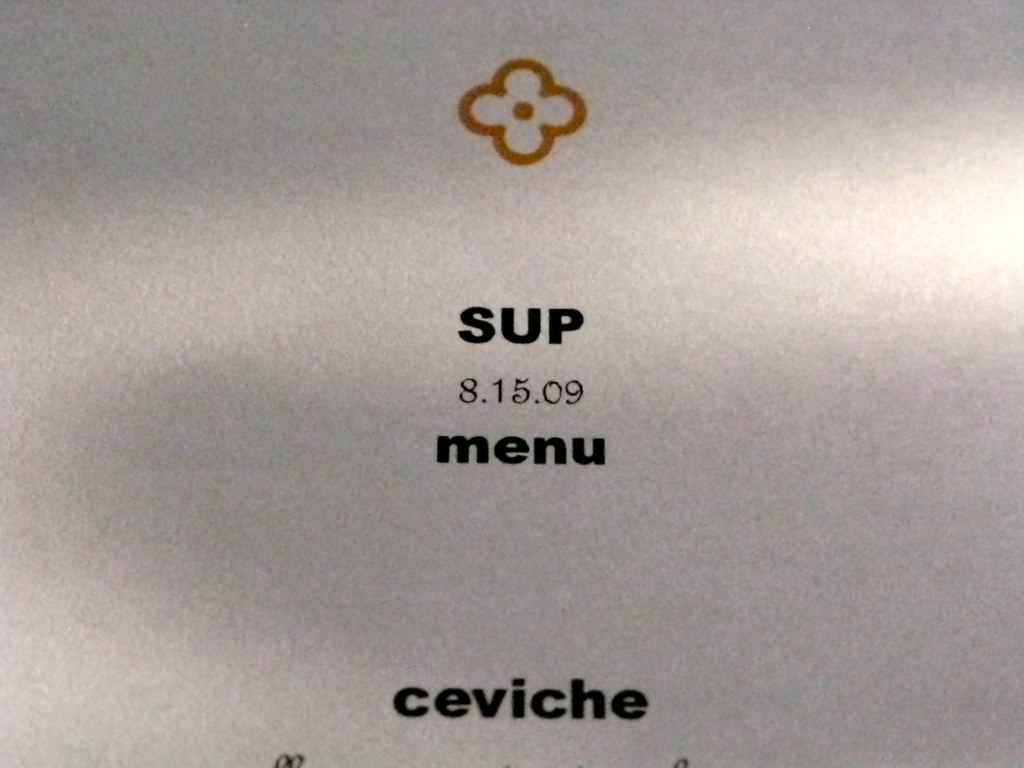A close-up image of a restaurant menu with a minimalist design featuring a grayish-white background. At the top of the menu, there is a gold four-leaf clover emblem reminiscent of the Louis Vuitton logo. Centered on the menu in bold, uppercase letters is "S-U-P" followed by the date "8-15-2009." Directly below this in smaller, black, lowercase letters is the word "menu." Towards the bottom center of the image, "ceviche" is written in black, lowercase letters. The photograph hints at additional text at the very bottom, which is partially cut off and only displays a few indistinct loops.